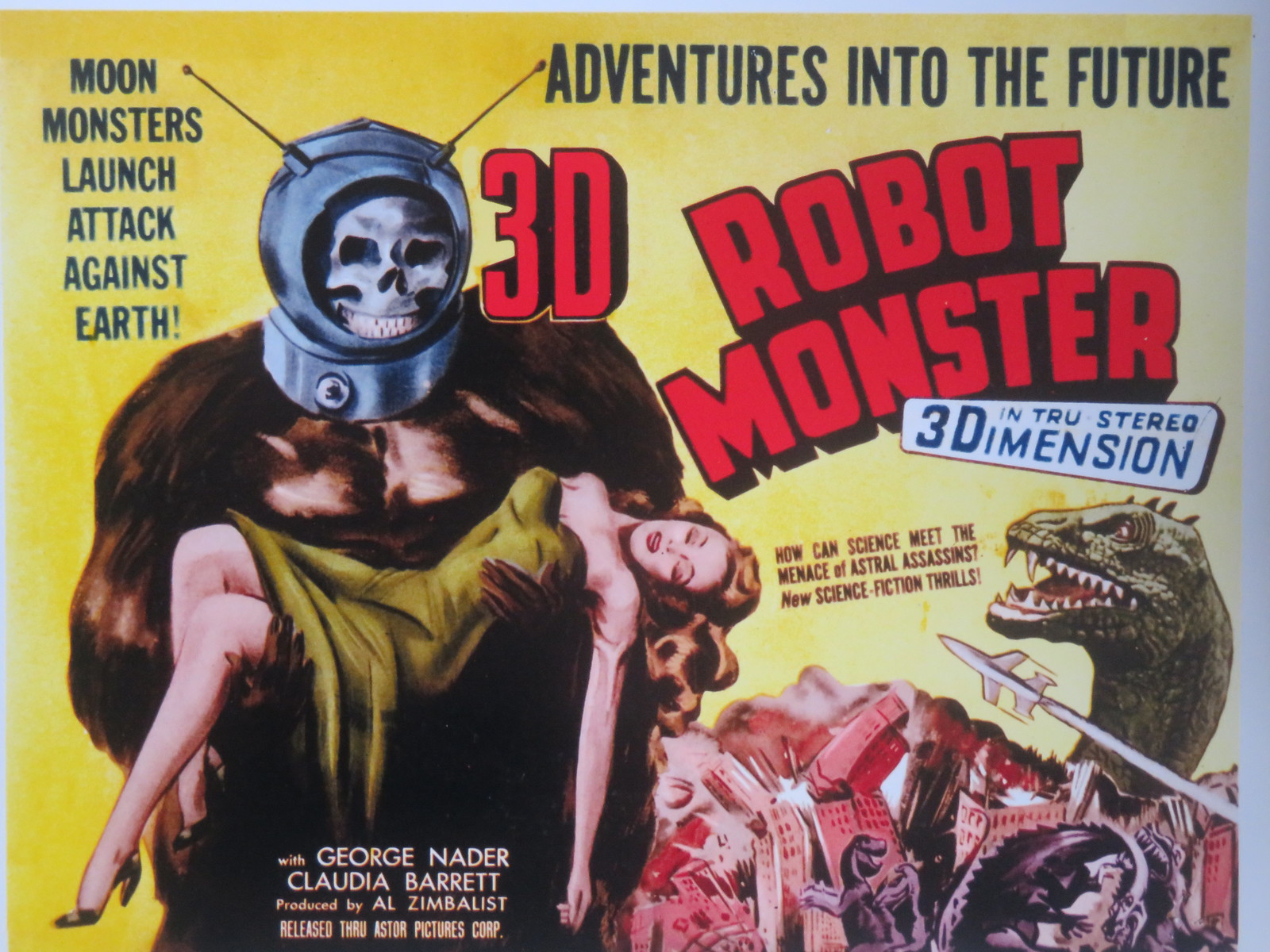This vintage movie poster, set against a striking yellow background, showcases a dramatic advertisement for a science fiction thriller. Dominating the left side is a menacing gorilla-like creature equipped with an astronaut helmet, within which a human skull is visible. The beast clutches a fainted woman in a green cocktail dress, her red hair cascading down. The title "3D Robot Monster" is prominently displayed in large red text, emphasizing its presentation in "true stereo dimension" and "3D." Below this, phrases like "Adventures into the Future," "Moon Monsters Launch Attack Against Earth," and "How Can Science Meet the Menace of Astral Assassins" further intrigue viewers with promises of new science fiction thrills. To the right, an angry dinosaur and another lizard-like monster are depicted attacking a crumbling city, with skyscrapers collapsing amidst the chaos. The poster also lists stars George Nader and Claudia Barrett, noting production by Al Zimbalist and its release through Astro Pictures Corp. This vividly painted scene encapsulates the sensational and apocalyptic themes typical of classic sci-fi cinema.